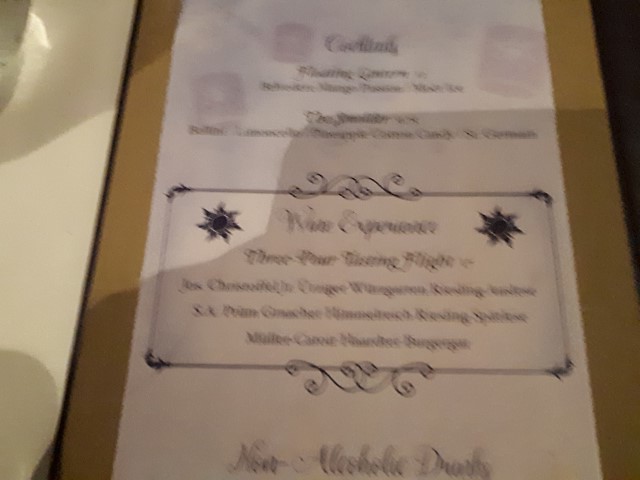A blurry photograph shows a white invitation page with torn, perforated edges. The centerpiece of the invitation features the words "Wine Experience" flanked by two stars on each side, though the text is somewhat difficult to read due to the image's lack of clarity. Further down, the text appears to mention a three-hour wine flight and includes some reference to Courtland. The bottom section of the invitation seems to advertise non-alcoholic drafts, but the blurred quality makes it hard to decipher the exact wording. The motion blur indicates the camera was moving when the picture was taken, adding to the overall difficulty in reading the finer details.